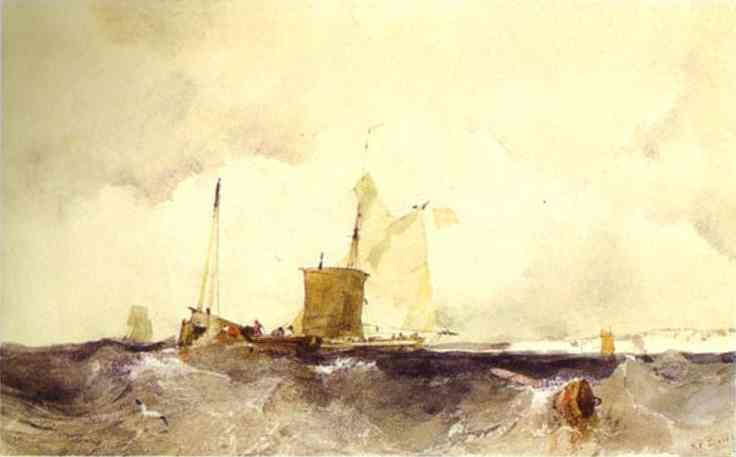This horizontally aligned rectangular painting, absent of any border, prominently features a turbulent seascape dominated by a vast, cloudy sky occupying the upper two-thirds of the image. The sky is a mix of beige, gray, brown, and a faint greenish tinge, with darker cloud formations concentrated more heavily in the top left corner. The bottom portion of the painting vividly illustrates wavy water, where the tips of the waves appear white against the brownish-blue ocean. The water also tinges with shades of purple and green, adding depth to the scene.

Centrally located in the painting is a ship, or perhaps a sailboat, characterized by its brown hull and white sails, complete with a flag fluttering. On closer inspection, an outline of a person, possibly a woman in a dress, is faintly visible on the vessel. Further left and slightly above the main ship is a smaller ship with a greenish-yellow square sail. The detailed depiction suggests it might be involved in some sort of maritime activity, potentially even a battle scene given the turbulent waves.

Adding to the narrative in the bottom right portion of the image is a greenish-reddish object, possibly a bucket or barrel, suggesting elements of a rough sea environment. The entire scene exudes an atmosphere of impending storm or ongoing maritime struggle, with the crashing waves and cloudy skies creating a dramatic and dynamic composition.